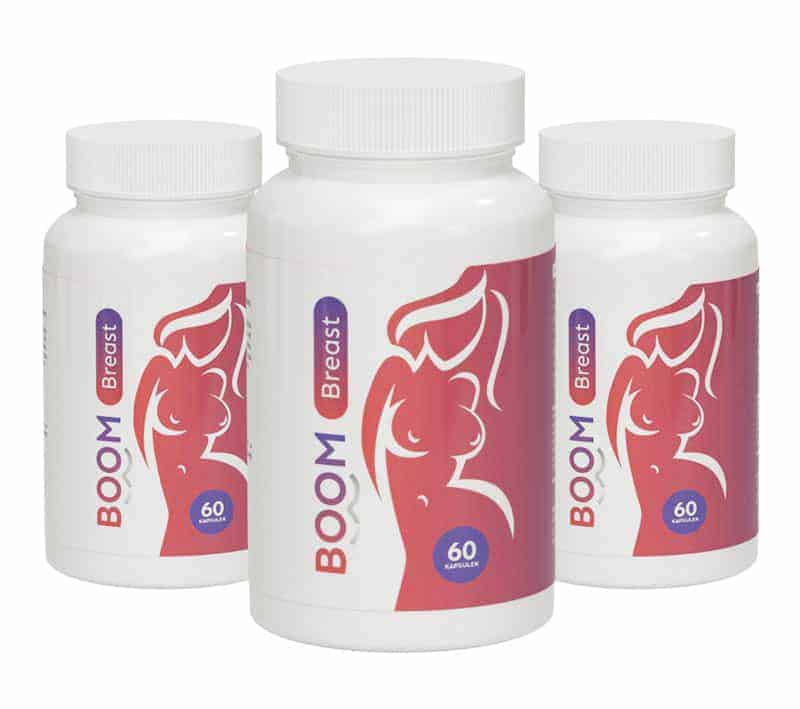The image depicts three identical white pill bottles arranged to form a triangle, with one larger bottle prominently in the foreground and two slightly cut off bottles in the background. The entire scene is set against a plain white background, typical of a stock image or advertisement. Each bottle is labeled "Boom Breast" and contains 60 capsules. The design on the bottles features a red-to-purple gradient, with the word "Boom" transitioning from red to purple, and "Breast" written in white letters within a capsule graphic. Additionally, there’s a simplistic, cartoon-style silhouette of a naked woman on the right side of the label, characterized by prominent, detailed breasts and facing to the right. A blue circle near her abdomen area further highlights the number "60" to indicate the pill count.